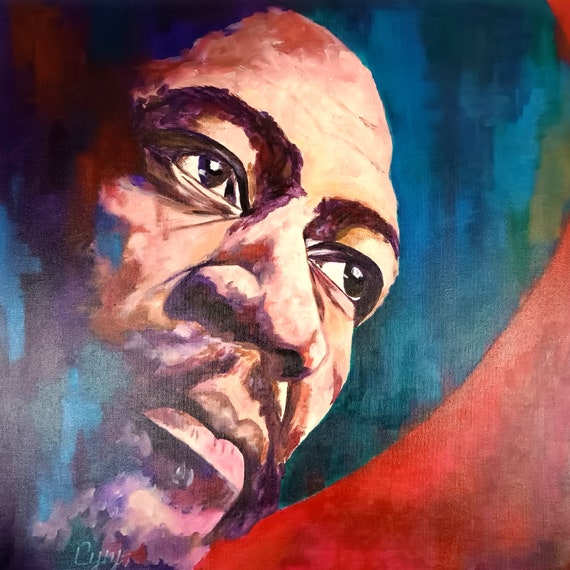This image is a detailed watercolor painting of an African American man's face, with an artsy and splotchy design. The man's face is angled from the upper middle to the lower left corner. He looks serious and is looking to the right, while the right-hand side of his face fades into an abstract blend of dark blue, red, and light blue colors. The background is a dynamic mix of blue and green shades, with a distinctive red, arched triangle in the lower left. His skin tone is depicted using various colors, including blue-green, purples, and blues, creating shadows on his face. Dark eyebrows and a slightly brown mustache are visible, and he has what appears to be an afro. There is also some illegible text at the bottom left, possibly the artist’s signature.